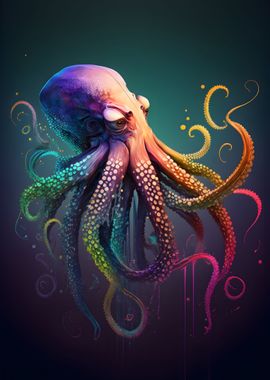This image is a detailed and vibrant artwork of an anthropomorphic octopus, floating in a lush blue-green sea. The octopus is depicted in a rainbow of colors, with a body predominantly whitish and magenta. It has large, expressive eyes adorned with eyelids and eyelashes, lending it a whimsical, almost human-like quality. The octopus is illustrated with multicolored tentacles, each arm showcasing a blend of hues; some tentacles start off in shades of purple and transition into green, while others are a mix of pink, fuchsia, blue, and lime green. The octopus is positioned facing to the right, with its tentacles curling and splaying out in all directions, capturing a sense of dynamic movement. The overall impression is of a fantastical and richly saturated underwater scene, encased in a dark bluish-gray rectangular frame.